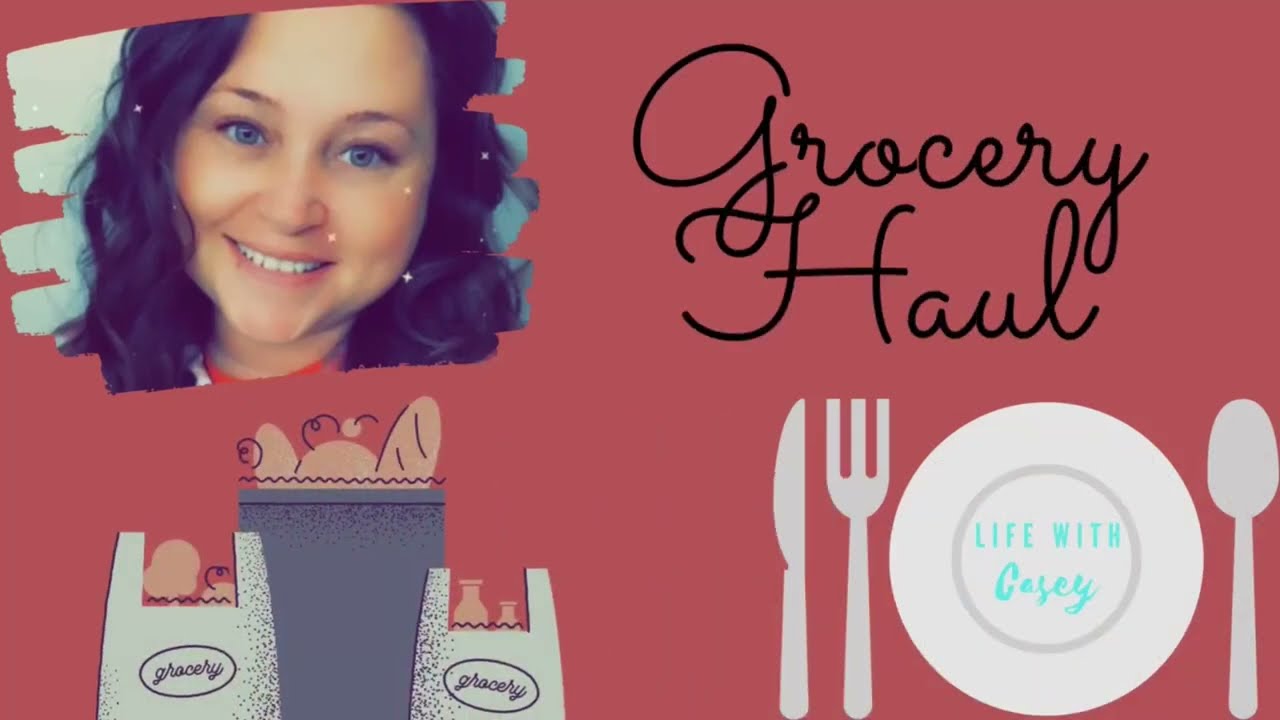This image is a vibrant title card featuring a mixed-media design with a photograph of a smiling woman and various graphic elements. The background is a rich red color, providing a striking contrast to the other elements. Positioned on the upper left-hand side of the image is a close-up photo of a woman with long, wavy brown hair and blue eyes. She appears to be around one to two feet from the camera and her picture has been enhanced with a filtering app to smooth out surfaces and brighten the colors.

Adjacent to her image, on the upper right side, is the phrase "Grocery Haul" written in black cursive font. Below this text, there is a silver silhouette of a knife, a fork, and a spoon surrounding a white plate. Inside the plate, in blue script, it reads "Life with Casey." Also present are graphical depictions of grocery bags containing brown icons of bread and bottles, aligning with the theme of groceries.